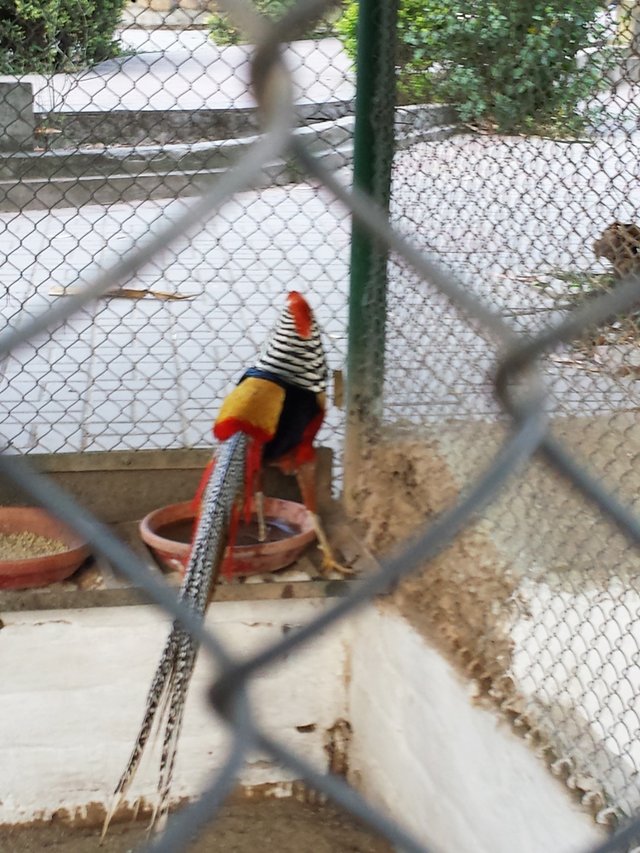The image features a striking and exotic bird, possibly a tropical species, inside a dingy, fenced-in cage. The bird is standing on a dirty ledge that holds two ceramic dishes, one of which contains water, while the other one is likely for food. The colorful bird, which resembles a rooster, has an intricate plumage: a very long tail with distinct black and white speckled feathers that taper to a point, and vibrant orange and red feathers on its bright back. It boasts horizontal black and white stripes from its shoulders to its head, crowned with a prominent red comb. Its strong, muscular legs are prominently positioned with one foot in the water dish and one outside. The bird faces away from the camera, gazing through the chain link fence into a sunny outdoor courtyard that includes a cement or stone drive, some plants, and stepped concrete structures in the background. The foreground is dominated by an out-of-focus chain link fence, through which the photograph is taken, adding to the sense of confinement within the cage.